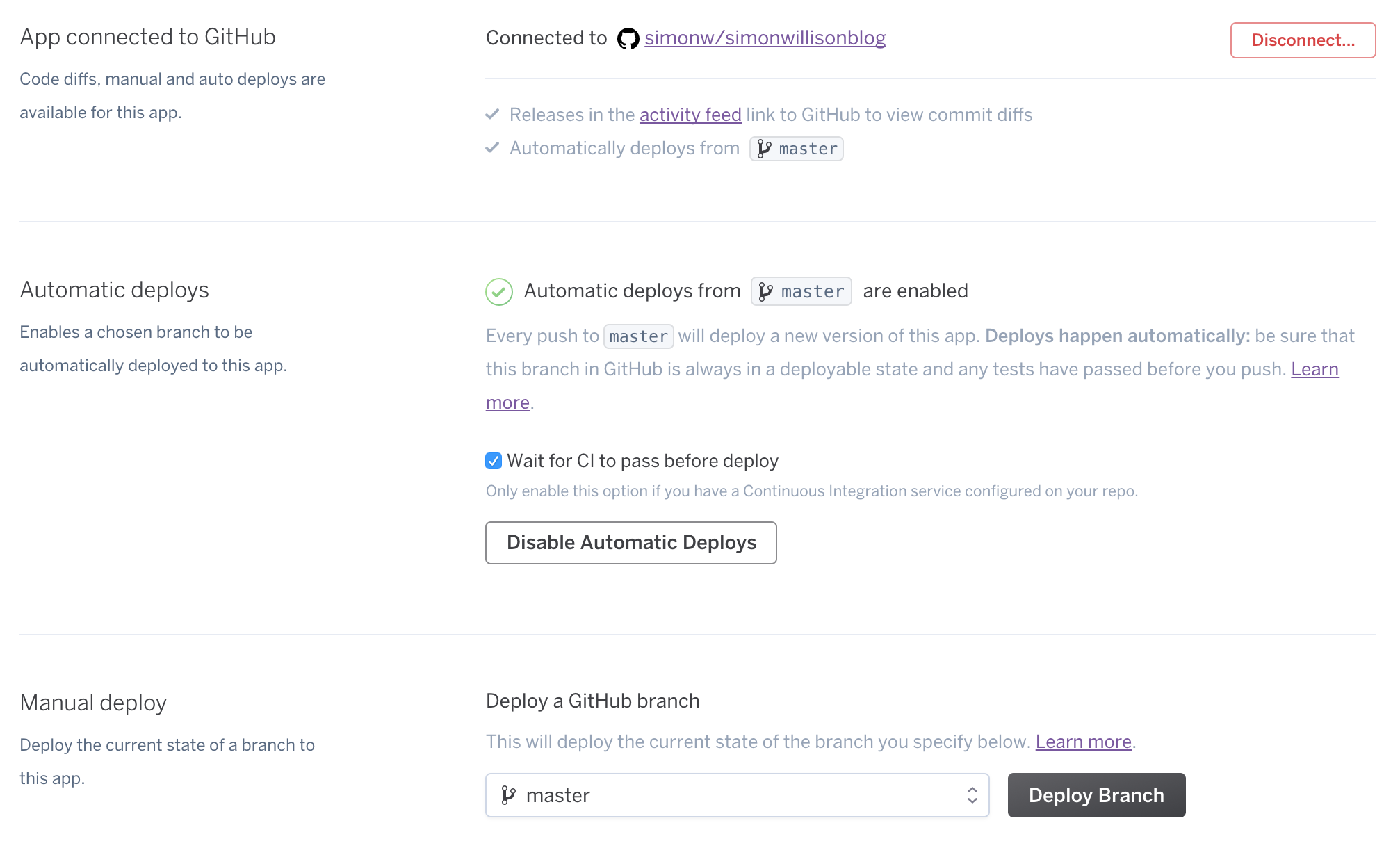Image Caption: A GitHub application interface is displayed, highlighting various features essential for collaborative software development. On the left pane, several sections are organized, including options for connecting the app to GitHub, viewing code differences, and setting up both manual and automatic deployments. The right side showcases the user's profile along with the application's URL. Detailed information about commits, deploys, and the status of the master branch is prominently featured. An automatic deployment section indicates that automatic deploys from the master branch are enabled and includes a checkbox to wait for CI (Continuous Integration) to pass before deployment. There's also a section for manual deployment, allowing the current state of the branch to be deployed from a dropdown, where the master branch is selected as the default. This setup is crucial for managing contributions from multiple developers who are working simultaneously on various branches of the same project. The interface features a clean, white background with black text and includes a 'Disconnect' button in the top right corner.